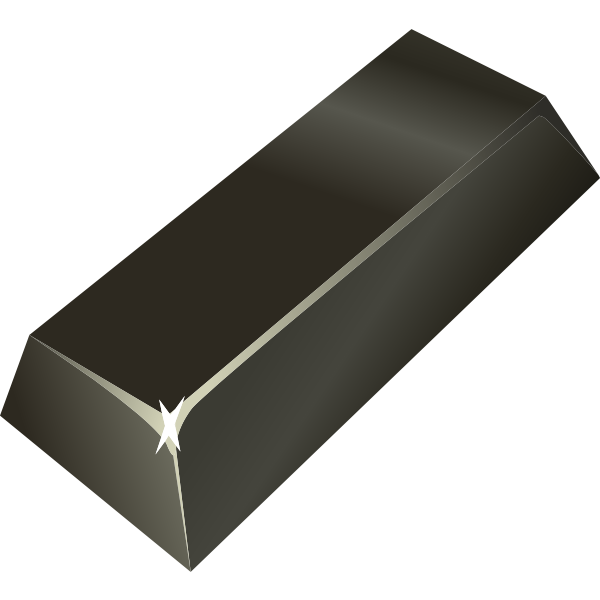The image showcases a three-dimensional, trapezoidal-shaped object positioned diagonally from the upper right to the lower left corner. The object appears to be metallic, predominantly gray-silver with elements of dark gray or charcoal coloring, and has reflective surfaces that suggest a shinier finish in certain spots to enhance its 3D appearance. The top face of the shape is black, transitioning to lighter shades along the edges. The object’s front-facing trapezoidal shape is outlined in silver, separating it from the top and sides, adding depth to the structure. There is a notable white, four-pointed star or X located at the corner closest to the viewer, giving a highlighted effect. The background is solid white, devoid of any additional text or elements. Overall, the shape resembles a block from a candy bar or a conceptualized gold brick, suggesting heaviness and a larger size than it might first appear.